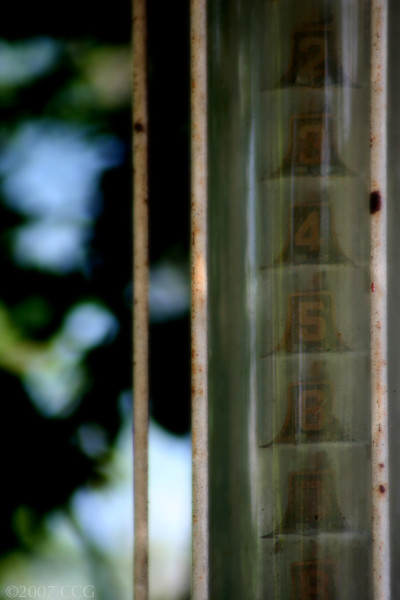This photograph features a glass cylinder encasing three vertical, white metal rods that exhibit a rusty, weathered appearance. Attached to these rods are small, bell-shaped flaps, each bearing a number. The sequence begins with the number 2 at the top, followed by numbers 3 through 8 in declining order. Each number is prominently displayed in white on the brown, rust-tinged flaps. The reflective surface of the curved glass cylinder further emphasizes its transparency and echoes the ambient light.

In the blurred background, silhouetted foliage contrasts against a brightly illuminated sky, suggesting daylight. Hints of green beyond the silhouette indicate additional layers of vegetation. The sky that peers through the foliage is a vibrant blue, adding a serene backdrop to the rustic object in the foreground.